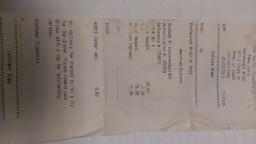The image is a low-resolution, landscape-oriented color photograph of an old, off-white receipt, creased and folded lengthwise. The receipt is positioned horizontally, requiring a 90-degree clockwise rotation to be read correctly. The writing, though unclear and rendered in a dark grey or bluish ink, features several distinct sections separated by lines. The top section likely contains store or restaurant information, followed by sections detailing the items purchased and their prices. A horizontal line further down may denote spaces for tax, tip, total, and a signature line marked with an X. The background appears to be a marble-style countertop with grey striations, contrasting slightly with the receipt’s aged, yellowed paper. Despite the fine details being illegible, the overall structure and purpose of the receipt as a record of a transaction are still discernible.